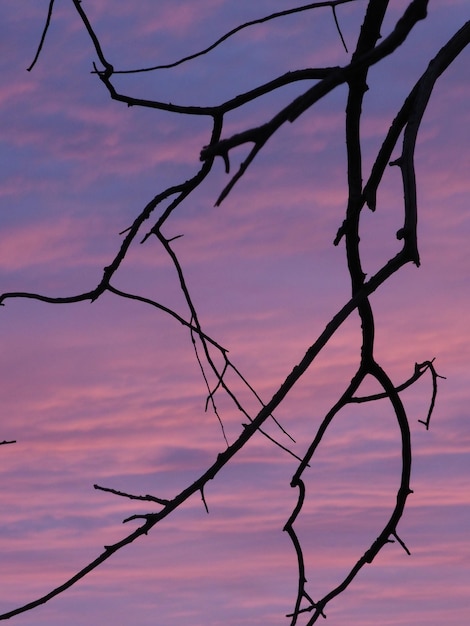The image is a detailed, up-close silhouette of a spindly, barren tree set against a stunning dusk sky. The foreground features the intricate, twisty branches of the tree, appearing almost black and resembling the sharp, fragmented lines of a broken mirror. These branches, devoid of any leaves, weave and criss-cross over each other, adding a textured, artsy feel to the scene.

In the background, the sky is a beautiful blend of delicate, hazy tones in purple, pink, and blue, reminiscent of cotton candy. The sun has nearly set, casting the scene in a soft, muted light. Puffy clouds fill the sky, adding layers of texture and interest, while areas of deeper blue hint at the encroaching night. There's no ground visible in the picture, which accentuates the stark, dramatic contrast between the dark, bare branches and the colorful, cloud-strewn sky, creating a mesmerizing, almost surreal visual experience.